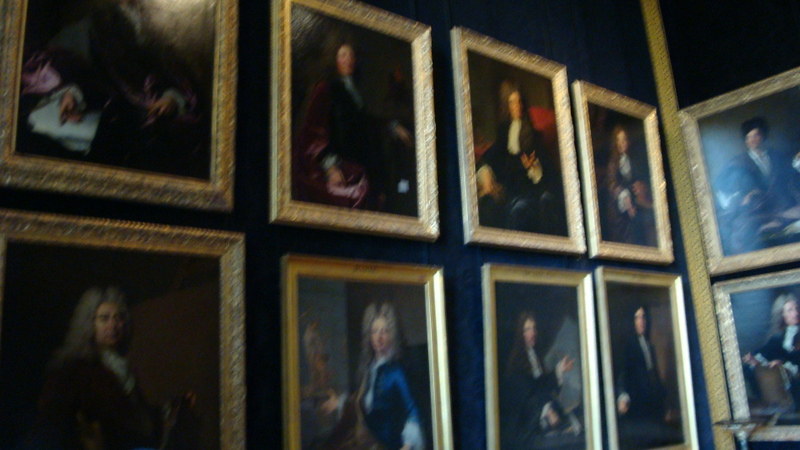The image depicts a collection of classical portraits displayed on the blue walls of a corner room, showcasing a total of 10 paintings. Each portrait is encased in an elaborate gold frame with intricate accents. The artworks appear to be formal, realistic depictions of older men, possibly from the 16th to 18th centuries, dressed in professional attire, including powdered wigs. The portrait subjects vary in their poses, with one man depicted reading papers in the top left corner, while the others are seated, gazing outward. The arrangement includes two rows of four paintings on the left wall, aligned evenly, and two additional paintings positioned vertically on the adjacent wall. The cohesive display exudes an air of historical significance, possibly representing figures of authority such as past presidents or government officials. The blue walls create a distinguished backdrop that highlights the golden accents of the frames, enhancing the classic elegance of the scene.